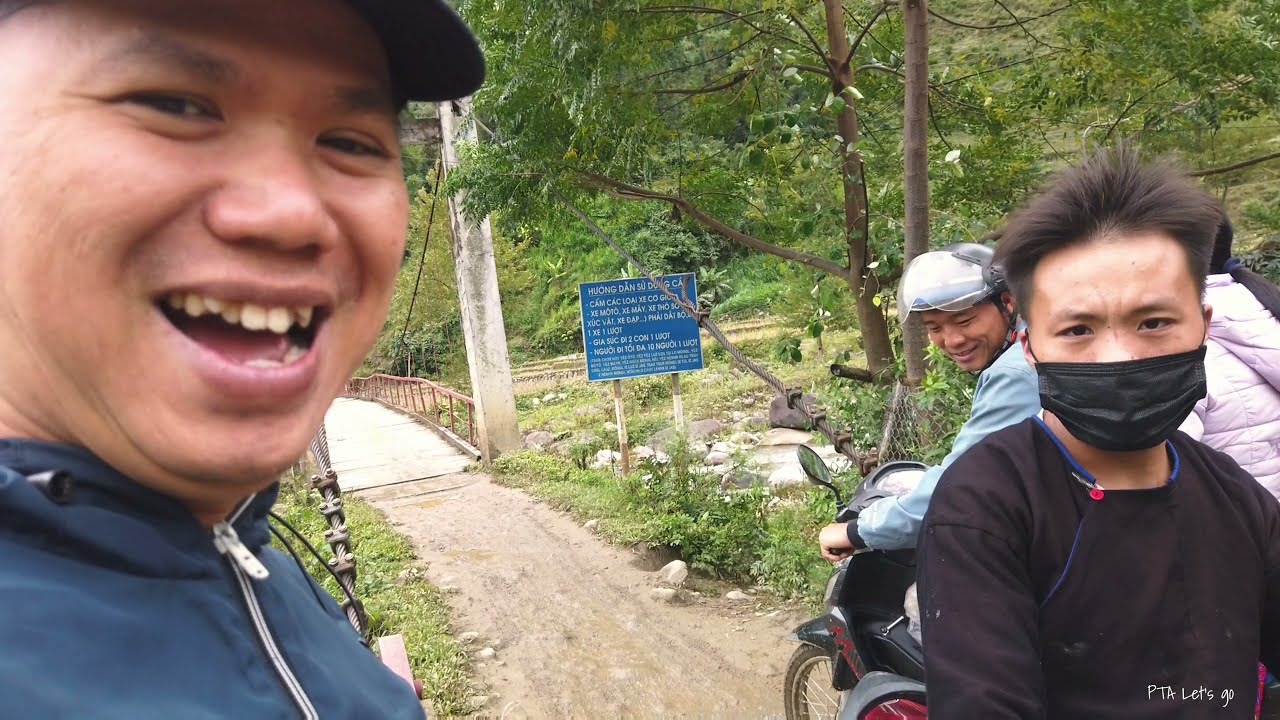In this detailed outdoor scene, a group of individuals is captured in a selfie taken by a man on the left. He dominates the frame, wearing a black billed hat and a blue zip-up jacket, smiling broadly with his mouth open, revealing his crooked teeth. To his right, in the front, stands a man with short, spiky brown hair, wearing a black shirt and a black COVID-style mask, his hair lifting as if in the wind. Directly behind the masked man, two people are on a black and red motorcycle. The driver has on a blue jacket and a gray helmet with a visor, slightly turned to look back. The passenger, partially obscured, wears a lavender coat. The background showcases a natural area with a dirt path leading to a concrete bridge. Shrubs, rocks, and green trees populate the scene. A blue sign, with text in an unrecognizable language, is near the center of the image. The only legible text in the photo, "PTA let’s go," is situated in the bottom right corner. The serene, verdant backdrop contrasts with the dynamic foreground action, creating a vivid exploration scene.